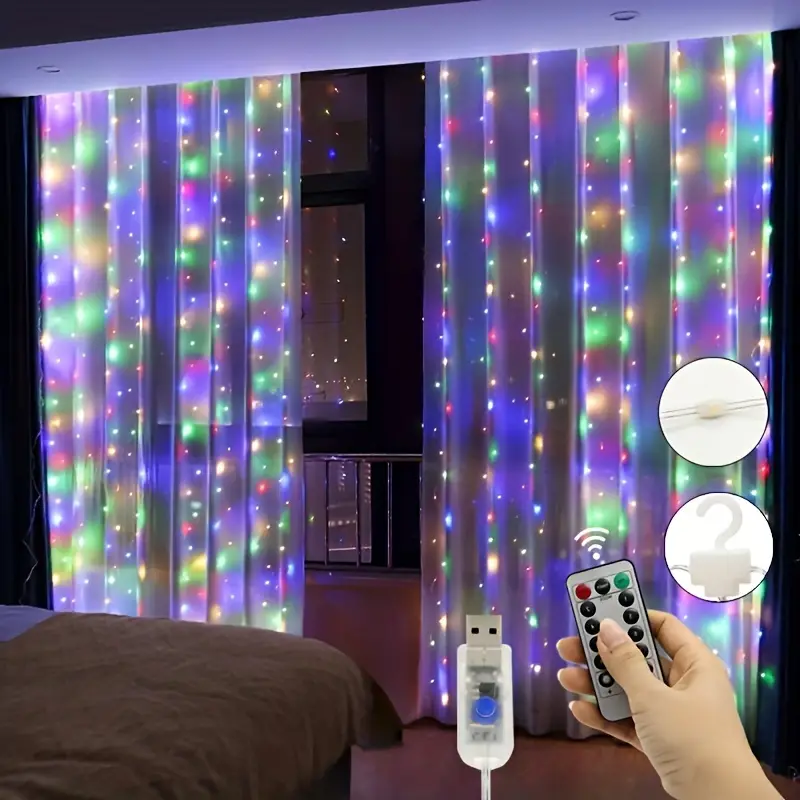This color photograph appears to be an advertisement showcasing a sophisticated bedroom setting in a high-rise apartment at nighttime. In the foreground, at the bottom left, a bed with a grayish blanket is visible. To the right, the focus is on a right hand holding a small, gray remote control with black buttons, a red button on the top left, and a green button on the top right. Above the hand are two white circles, potentially representing control mechanisms or decorative features, possibly superimposed for visual effect. Adjacent to the remote is a white, translucent USB port with a blue center and a translucent white cord trailing off it. 

The main subject of the photo is the set of sheer, translucent curtains embedded with rows of red, white, blue, and yellow strobe lights, creating a vibrant effect. These curtains are draped on the left and right sides of a large window or patio door, which opens to a city skyline, enhancing the perception of being high up. The remote in the hand suggests control over the LED light curtains, possibly to turn the lights on and off or to open and close the curtains. This image, with its various superimposed elements and detailed features, looks like an online product advertisement aimed at highlighting the functionality and aesthetic appeal of the smart curtains and their remote control system.